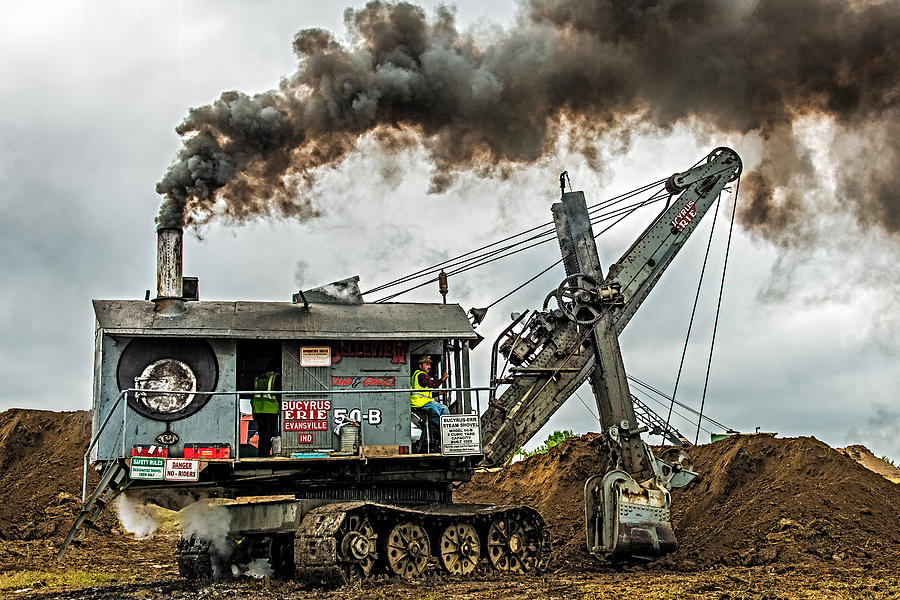This photograph, taken outdoors during the daytime, captures an old-fashioned steam shovel machine atop caterpillar treads, working amidst a large pile of brown dirt that spans the background. The machine, identified by its tracks with internal wheels allowing mobility, supports a rustic blue-gray wooden cabin with a slanted roof. A thick silver smokestack protrudes from the back of the cabin, belching thick black and gray smoke into the dark gray, cloud-covered sky.

On the front of the cabin, a small red sign with white text reads "Bucyrus Erie Evansville," highlighting the machine's make. Just past the sign, we see a rectangular doorway on the right end of the cabin, where a driver is visible, seated and operating the controls. Positioned centrally, another man stands in a doorway, further engaged with the machinery.

To the right side of the shack, a complex assembly of levered machinery and an articulated crane arm extend outward. This apparatus is meticulously managed through an intricate network of cables and pulleys, culminating in a scoop that actively digs into the dirt pile, creating a fresh mound as it functions. The hue of the crane and scoop match the dark gray of the machinery, contrasting with the earthy tones of the dirt and the subtle blue-gray of the cabin.